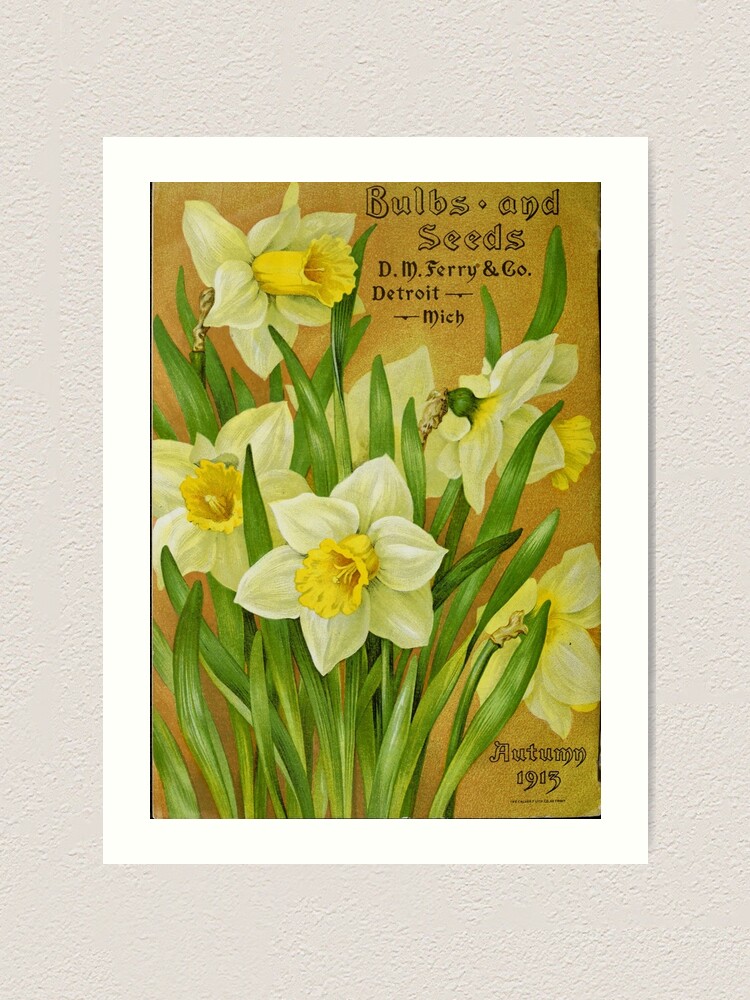This framed piece of artwork, set against a textured off-white wall, showcases a vintage seed packet adorned with five daffodil-like flowers. The white frame complements the delicate presentation of the flowers, which feature yellow cup-shaped centers surrounded by off-white petals. The flowers are intertwined with green leaves against a light tan background. At the top right of the artwork, elegant black lettering reads, "Bulbs and Seeds, D.M. Ferry & Co., Detroit, Michigan." Beneath the flowers, at the bottom right, is the inscription "Autumn 1915," accompanied by smaller, illegible text. The flowers are arranged in a way that displays various angles, with some flowers facing forward while others turn away, adding depth to the botanical illustration.